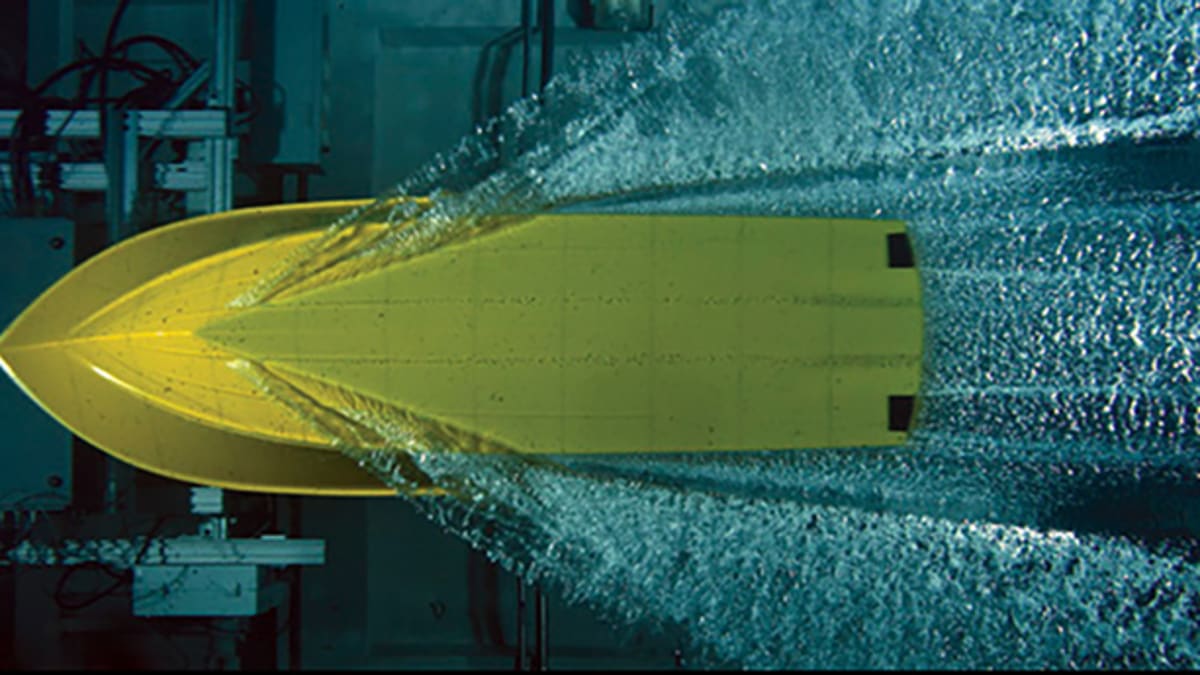The image depicts a rectangular photo primarily showing the top view of a yellow boat navigating through blue water. The boat, which occupies a significant portion of the photo's center, is moving from right to left, with its sharp, pointy bow facing the left side of the image and its lightly curved stern at the right. Two black squares are visible on the back of the boat—one positioned above the other. As the boat travels, it leaves a V-shaped wake in the water, with the V pointing towards the left side of the image. The background includes what appears to be mechanical equipment or fences, suggesting that the photo might be a scan or composite image, possibly taken at night.